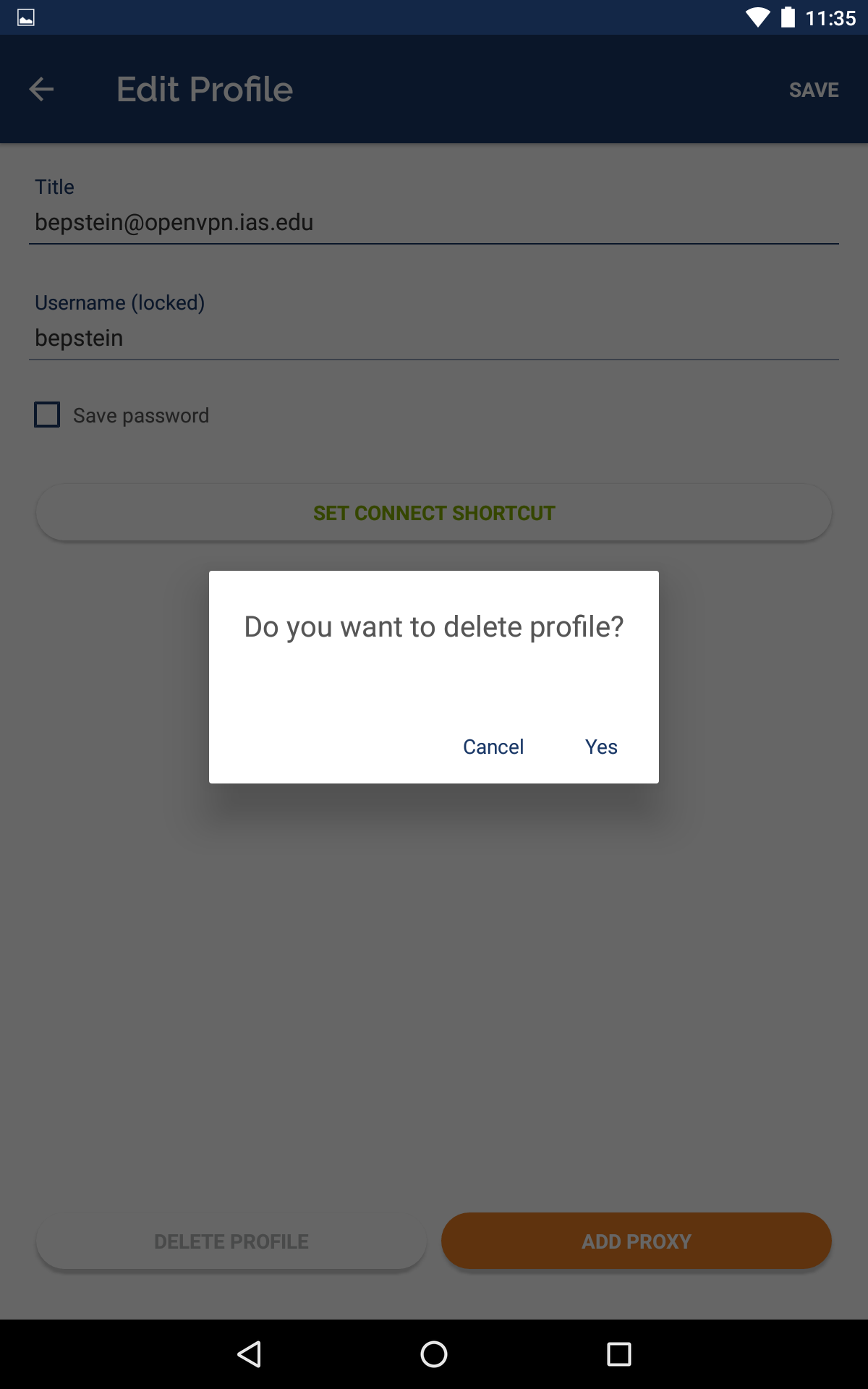The image is a color screenshot of a mobile phone taken at 11:35, though it's unclear whether it's AM or PM. The phone has a full battery and strong signal reception. At the bottom of the screen, there are three navigation buttons: a triangle pointing left (back button), a circle (home button), and a square (overview button). 

The screenshot displays an "Edit Profile" screen within an unidentified app, highlighted by a dark blue banner at the top with "Edit Profile" written in white text. The account being edited has the email address "bepstein@openvpn.ias.edu" and the username "BEPSTEIN." Two options are visible: "Save Password," which is not selected, and "Set Connect Shortcut."

The background is slightly dimmed, as a prominent dialog box in the center asks, "Do you want to delete profile?" with two options below: "Yes" or "Cancel." The user's next action, whether they will proceed with deleting the profile or cancel the request, is unknown.